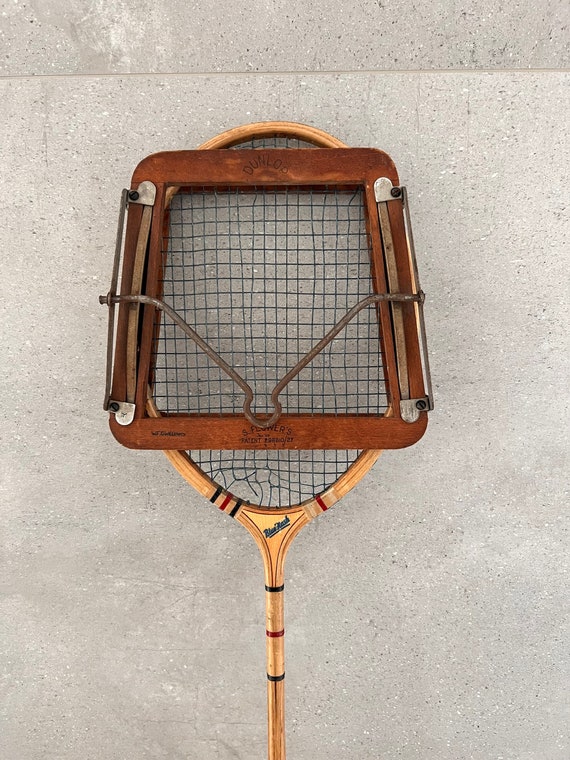The image showcases a close-up of an old wooden tennis racket, resting on a speckled concrete background. The racket itself is characterized by light-colored wood adorned with stripes at the handle—two navy blue stripes flank a central red stripe, adding to its vintage appeal. This well-used racket has evident signs of age, including a large hole in the bottom left part of its netting, with additional breaks in the strings, indicating extensive usage or wear and tear. Overlaying the racket's head is a dark cherry wood racket protector, designed to maintain the racket's shape and prevent warping. This protector, which isn’t quite a perfect square due to its angled sides, features metal brackets on the left and right edges and a central, bent metal bar that serves as a clamp. The brand name, possibly “Blue Flash,” is visible though obscured by age. This setup provides a nostalgic glimpse into how tennis equipment was carefully maintained in the past.